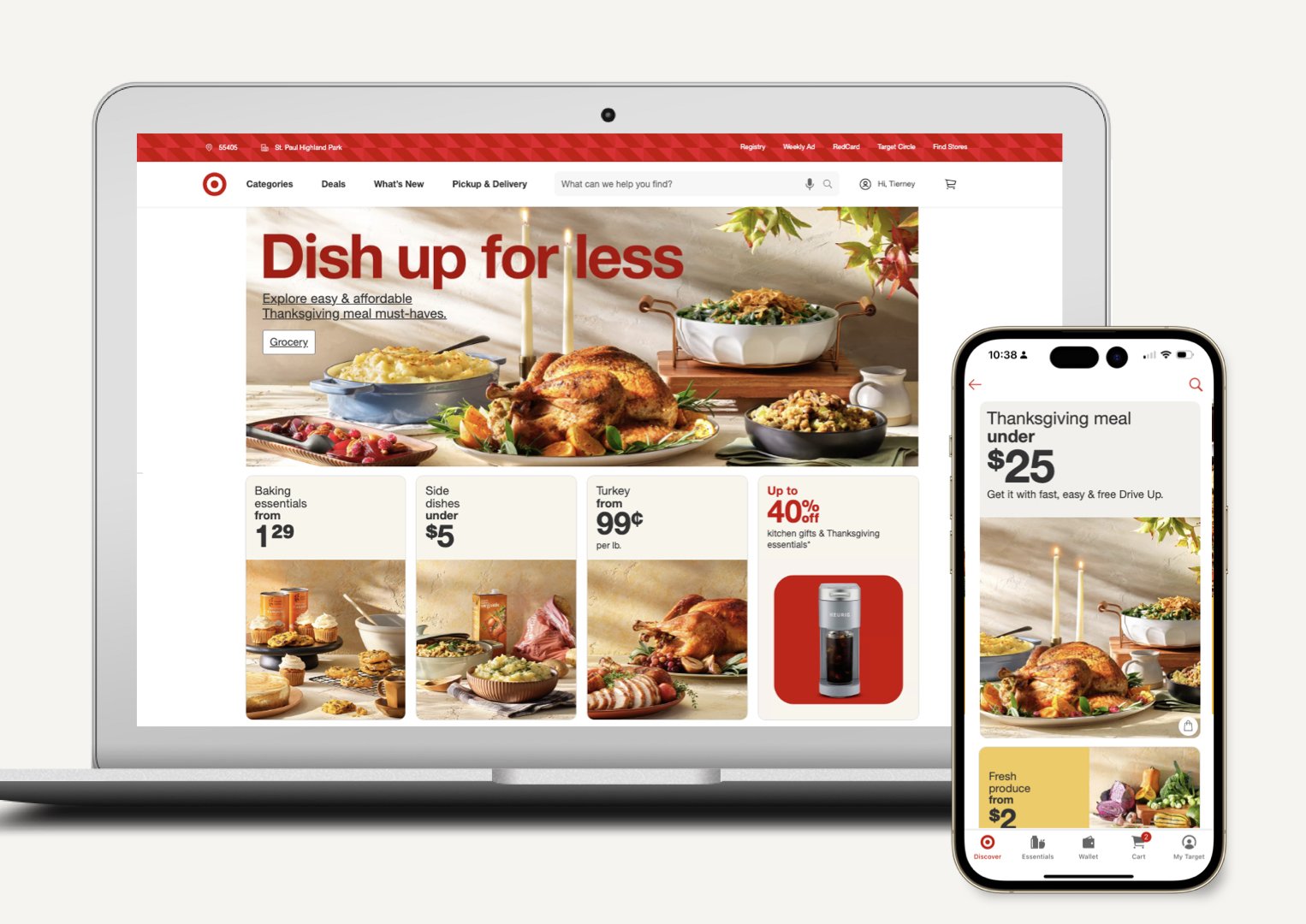The image displays a vibrant website designed for purchasing food and exploring recipes. At the top, a red banner stretches across the screen with small, hard-to-read text flanking both sides. Beneath the banner, bold and easily readable menu options are set against a white background, including categories for "Deals," "What's New," "Pickup and Delivery." The site clearly focuses on culinary products and meal preparation.

The central section of the webpage features an enticing image of a fully-prepared meal, starring a succulent turkey surrounded by bowls of various vegetables. Accompanying the image are promotional texts highlighting "Baking essentials from $1.29," "Side dishes under $5," "Turkey from $0.99 per pound," and significant discounts such as "Up to 40% off with a kitchen gift" and "Thanksgiving essentials."

Below the main image, there are four smaller pictures: one showcasing delicious desserts, another filled with fresh vegetables, a third displaying assorted meats, and the last featuring a refreshing glass of Coca-Cola. Adjacent to these images, a smartphone is depicted, displaying what appears to be the same deal shown on the laptop screen, featuring a Thanksgiving meal available for under $25. This dual presentation illustrates the website's responsive design, optimized for both desktop and mobile viewing experiences.